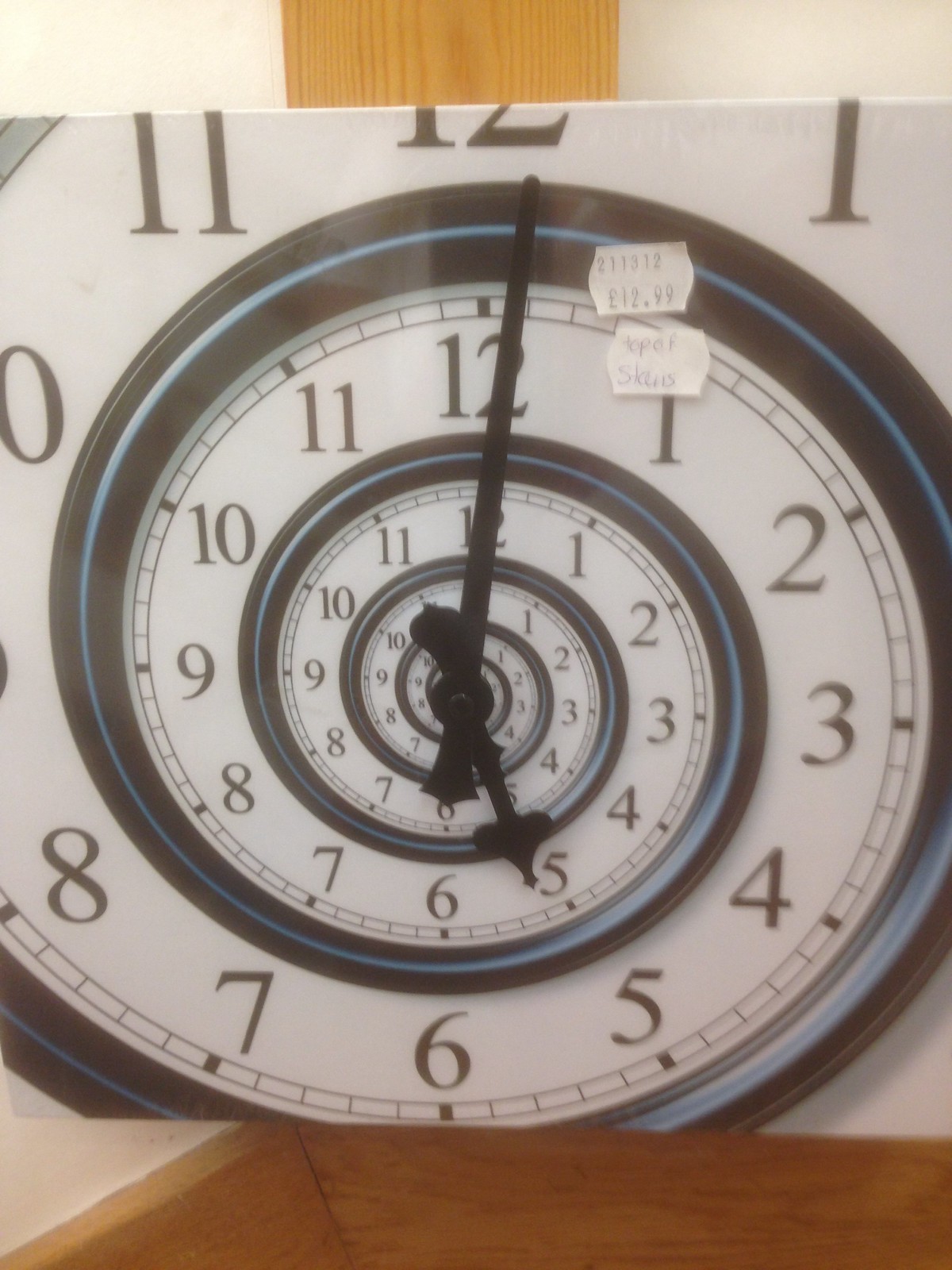This image features a modern, artistically painted clock with a white background. The clock face is adorned with intricate black swirls accented with subtle hints of blue, creating a dynamic and eye-catching design. Numbers 1 through 12 are displayed twice in bold black text on the clock. The artwork is propped up on a wooden easel. Two price tags are visible in the image; one is clearly marked at £12.99, suggesting a UK location. The second price tag is unreadable. The scene is devoid of people, allowing the focus to remain entirely on the unique clock.